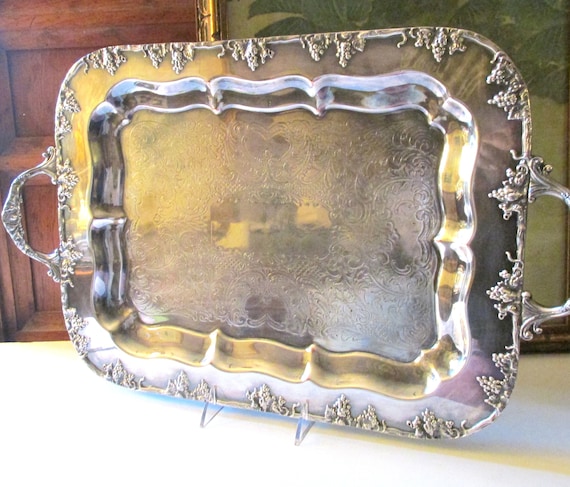The image showcases an ornate silver serving tray, positioned upright on a white table, supported by small metal stands beneath it. This polished silver tray, with its reflective finish, is intricately designed with a scalloped edge that forms gentle waves along its perimeter, adding a sophisticated touch to its overall shape. The edges of the tray are adorned with elaborate embossed patterns, featuring floral and grapevine motifs, providing a textured contrast to the smooth center. The handles, situated on the shorter ends, are embellished with similar designs, blending functionality with aesthetic appeal. The central area of the tray features detailed etching, with a non-etched oval section in the middle, enhancing its elegant appearance. The background consists of a brown wooden door to the left and a green painting partially visible on the right, suggesting the setting is inside a house.